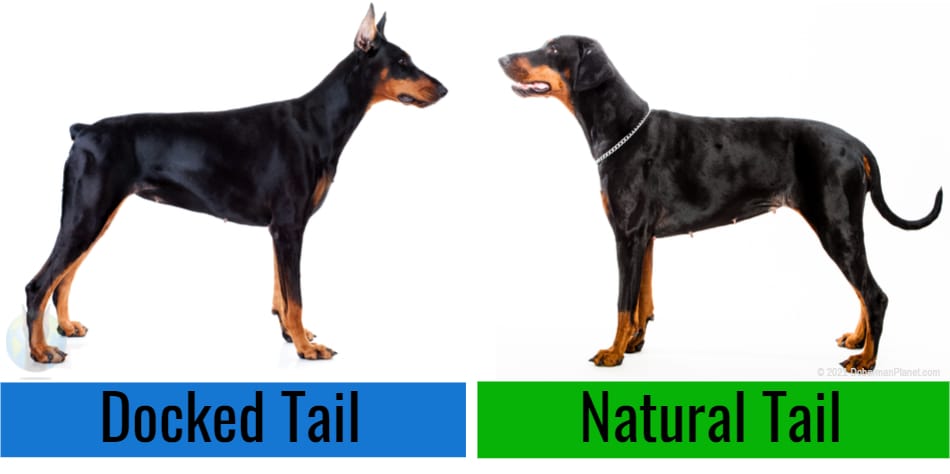The image appears to be an informational illustration, likely sourced from a textbook, displaying two Doberman Pinschers side by side to compare the physical differences between natural and altered states. Both dogs are depicted in full color, in silhouetted form, standing in profile facing each other. 

On the left, a Doberman with a docked tail and cropped ears is shown. This dog, identifiable by its rigid stance and erect ears, has a short, nubby tail and a black coat with brown markings on the paws and lower face. A prominent blue label beneath this image reads "docked tail."

To the right, a Doberman with a natural tail and uncropped ears is displayed. This dog, appearing more relaxed with its long, graceful tail and floppy ears, wears a chain collar and showcases the same black coat with brown accents. A green label beneath this figure states "natural tail."

The illustration's setting is plain, likely emphasizing the educational content by avoiding background distractions. There is some illegible text at the bottom of the image, suggesting further explanation not fully readable in this depiction. The overall composition highlights the contrast between the modified and natural appearances of this dog breed.